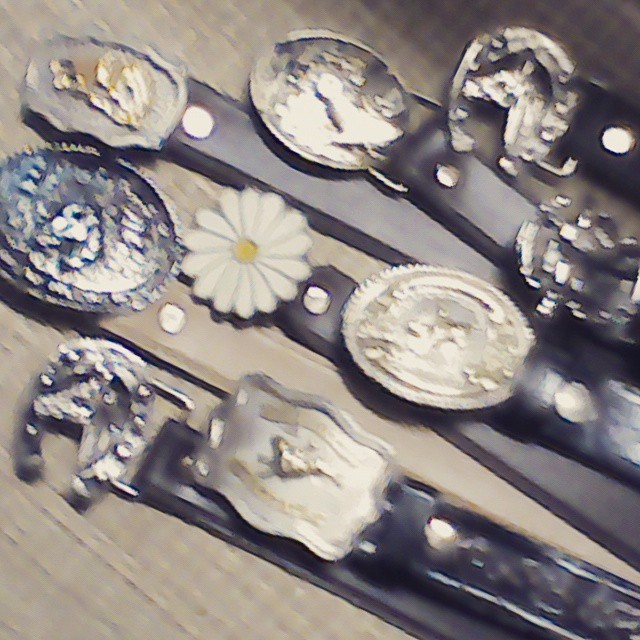The image displays an assortment of belt buckles laid out on what appears to be a brown wooden surface. Despite the overall blurriness of the photo, some details can be discerned. The buckles are of various shapes and sizes, including large ovals, smaller circles, and horseshoe designs. Many of them feature intricate designs, such as an image that seems to be a horse's head, although the blurriness makes it difficult to identify clearly. One notable buckle is designed like a daisy with white petals and a yellow center. Another buckle has a golden centerpiece framed by silver. Additionally, there's a round silver buckle with a blue tinge that possibly depicts a bird in the middle. The belts attached to these buckles appear to be primarily dark brown or black leather. The background is muted and has a textured look with horizontal and vertical lines, contributing to an impression of depth and softness despite the blur.